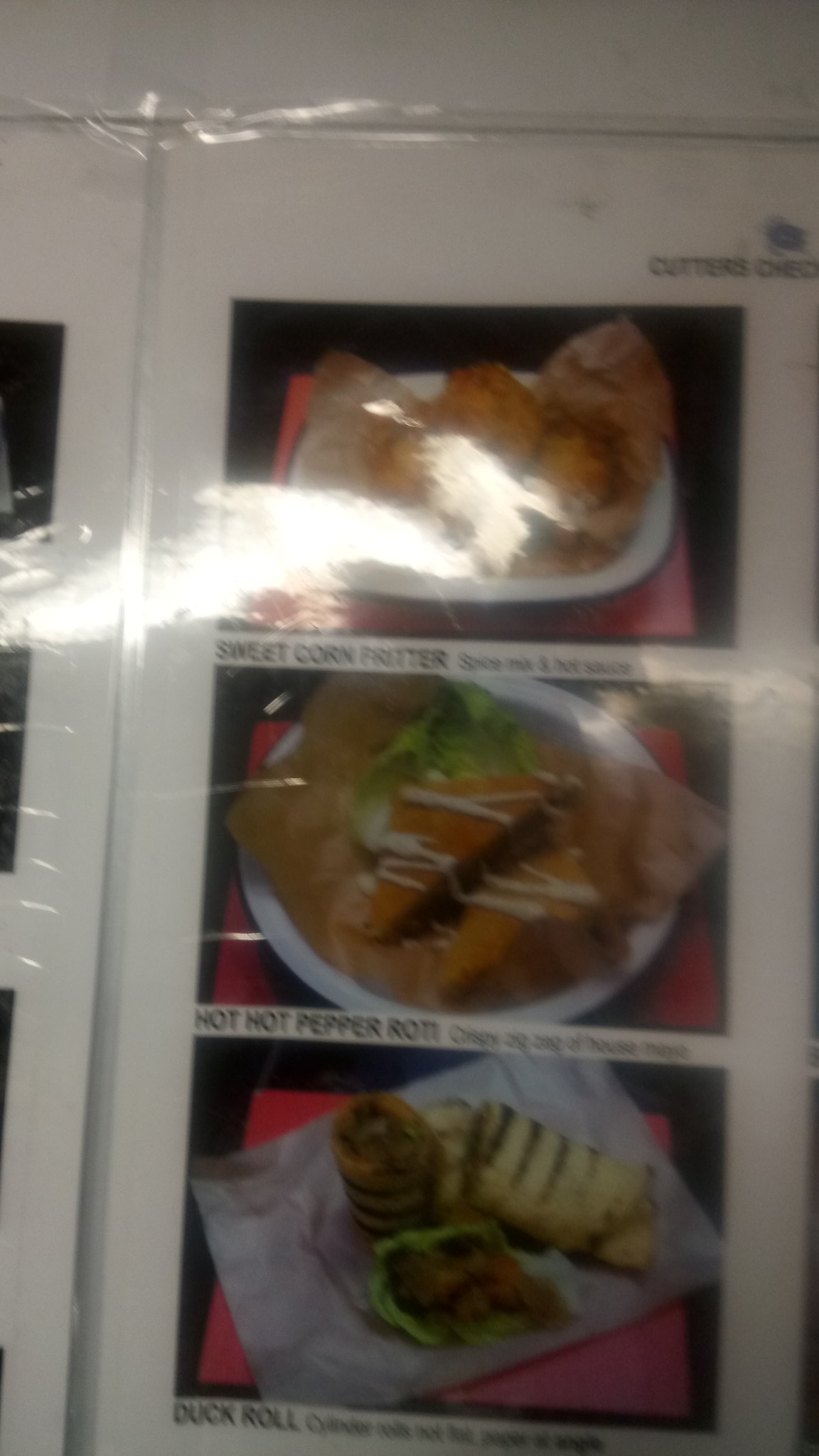This photograph captures a single laminated page of a restaurant menu, placed on a white surface. The low lighting and glare from the overhead light create a blurry effect and partially obscure parts of the menu. At the top right corner, in black letters, it appears to say "Cutter’s Check." The menu features three items, each accompanied by a photograph set against a red square tablecloth and a black background.

1. **Sweet Corn Fritter**: Described as containing spices and served with hot sauce, the image is partially obstructed by glare from the lamination.
   
2. **Hot Hot Pepper Roti**: The text describing this item is blurry, with only "crispy" discernible, making the rest of the description illegible.

3. **Duck Roll**: This item resembles a fatter version of an egg roll standing upright. The photograph also suffers from poor lighting, which hampers visibility.

Despite the low light and glare, the menu page provides a tempting glimpse into the offerings of this restaurant.